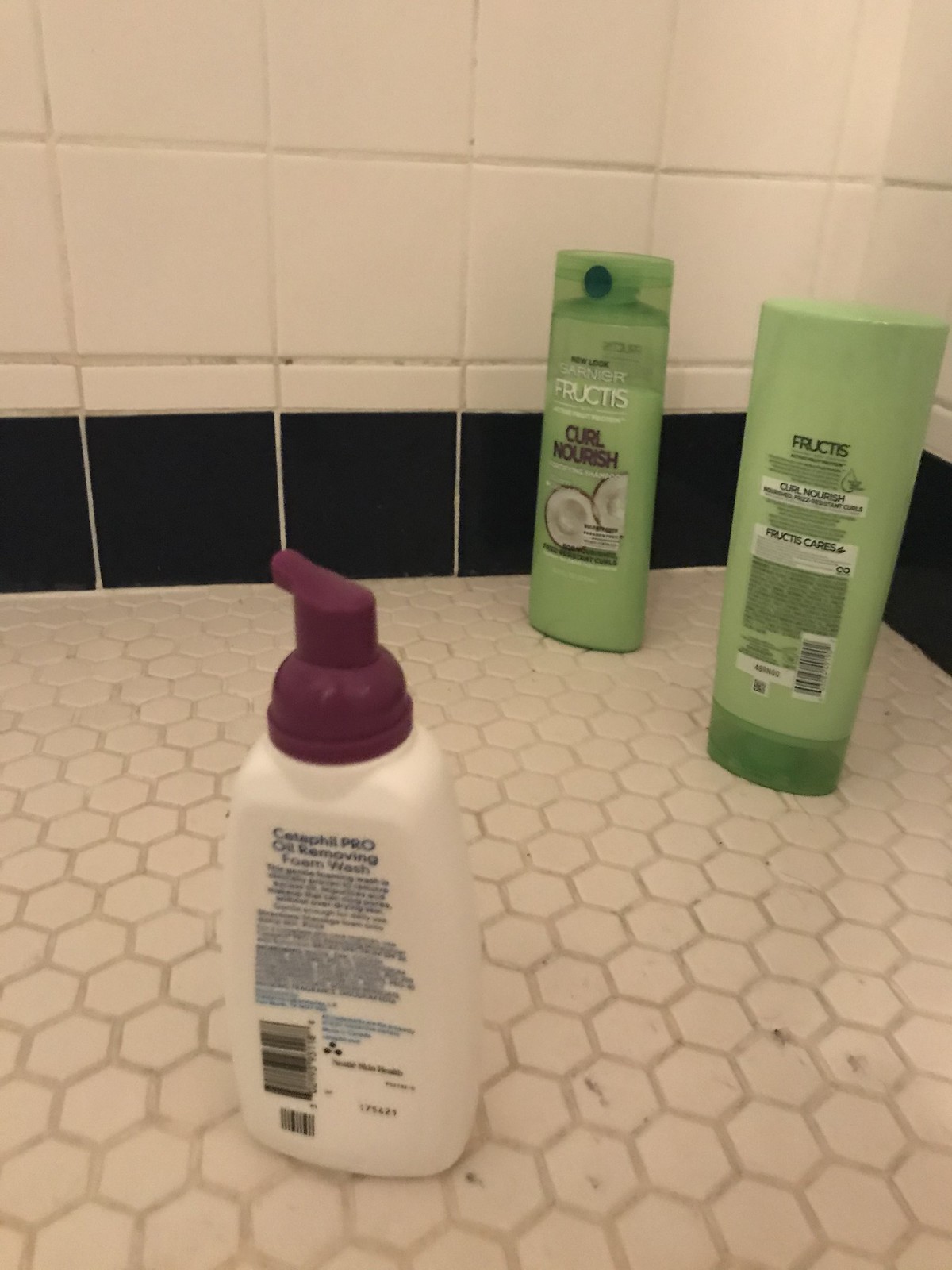This photo captures a close-up view of a bathroom floor or shower area, featuring a surface tiled with small hexagonal patterns. Along the wall, a white towel sits above a black towel placed at the tile base, adding layers of texture to the scene. The tiles on the walls are white with gray grout, accented by a border of square black tiles at the bottom. In the rear right corner, two green plastic tubes branded Fructus Curl Nourish are visible. One tube stands right side up, while the other lays upside down, possibly signaling recent use. Both tubes display an open coconut image on their labels. In the foreground, a white plastic container of Cetaphil Pro Oil Removing Foam Wash, with a dark purple pump, faces away from the camera, revealing the back of the bottle.